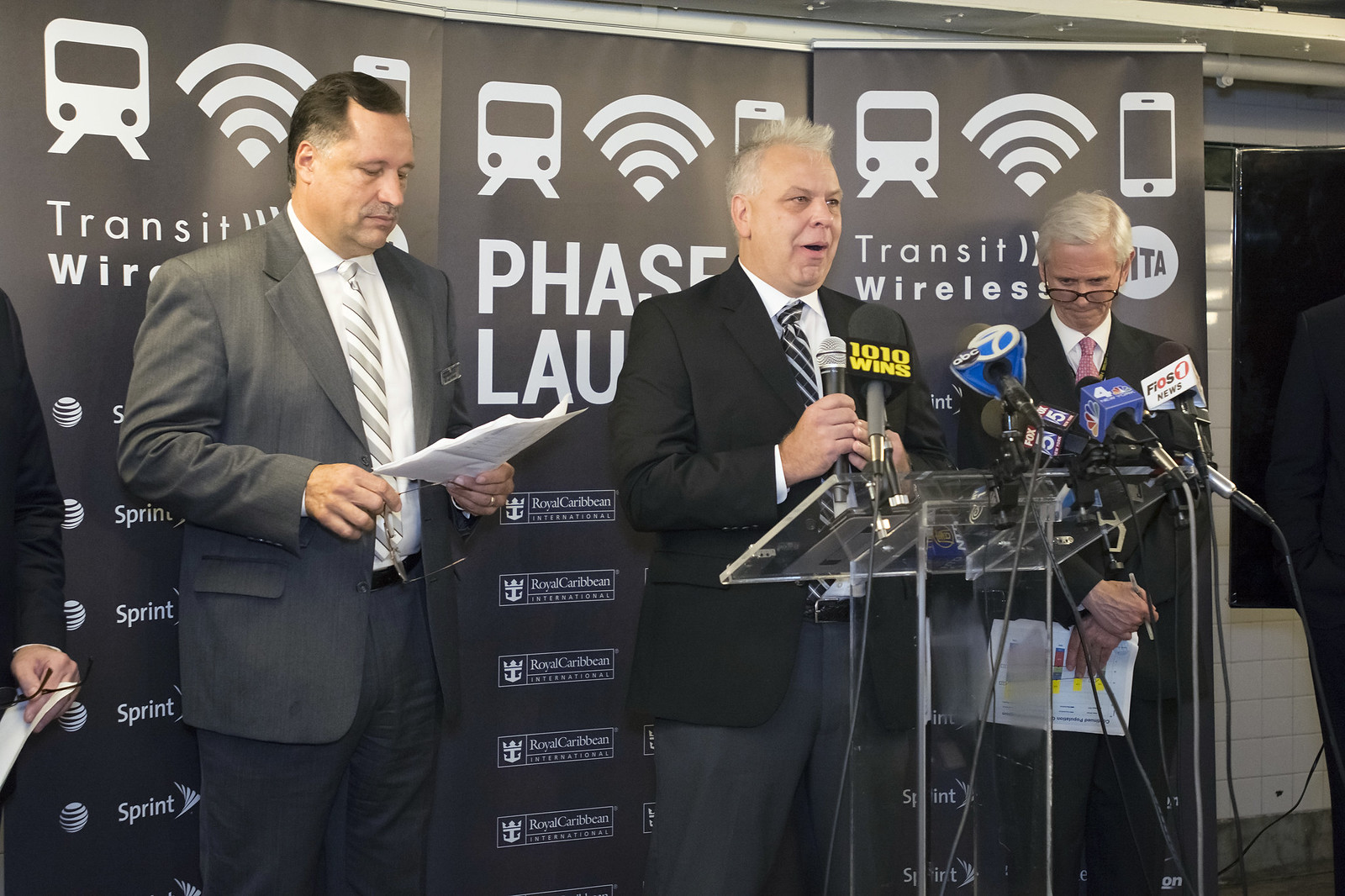The image is a landscape photo depicting a press conference with three middle-aged men standing prominently in front of a glass lectern. In the center is a man with short, slightly spiked gray hair, dressed in a black blazer, white collared shirt, and a black tie with white stripes. He appears to be speaking into multiple microphones from various news organizations, including ABC, NBC, Fox, and Fios 1 News, among others.

To his left, a man in a gray suit with a silver and white striped tie is looking down at a paper held in his left hand, while holding glasses in his right hand. This man has short black hair and appears to be intently focused on the document.

On the right, another man with gray hair and black glasses, worn low on his nose, is holding papers in his left hand and a pen in his right. He is dressed in a black suit, black pants, and a white shirt accompanied by a red tie with white polka dots. This man is slightly bent over, looking down at the lectern.

In the background, there is a black backdrop featuring various white symbols, including images of buses, Wi-Fi signals, and a cell phone. The backdrop includes partially visible text such as "Transit Wireless MTA," and logos for Royal Caribbean and Sprint, which contribute to the context of the event. The overall setting is well-lit, suggesting the use of natural lighting. The scene captures the formal atmosphere of a public announcement or press briefing.